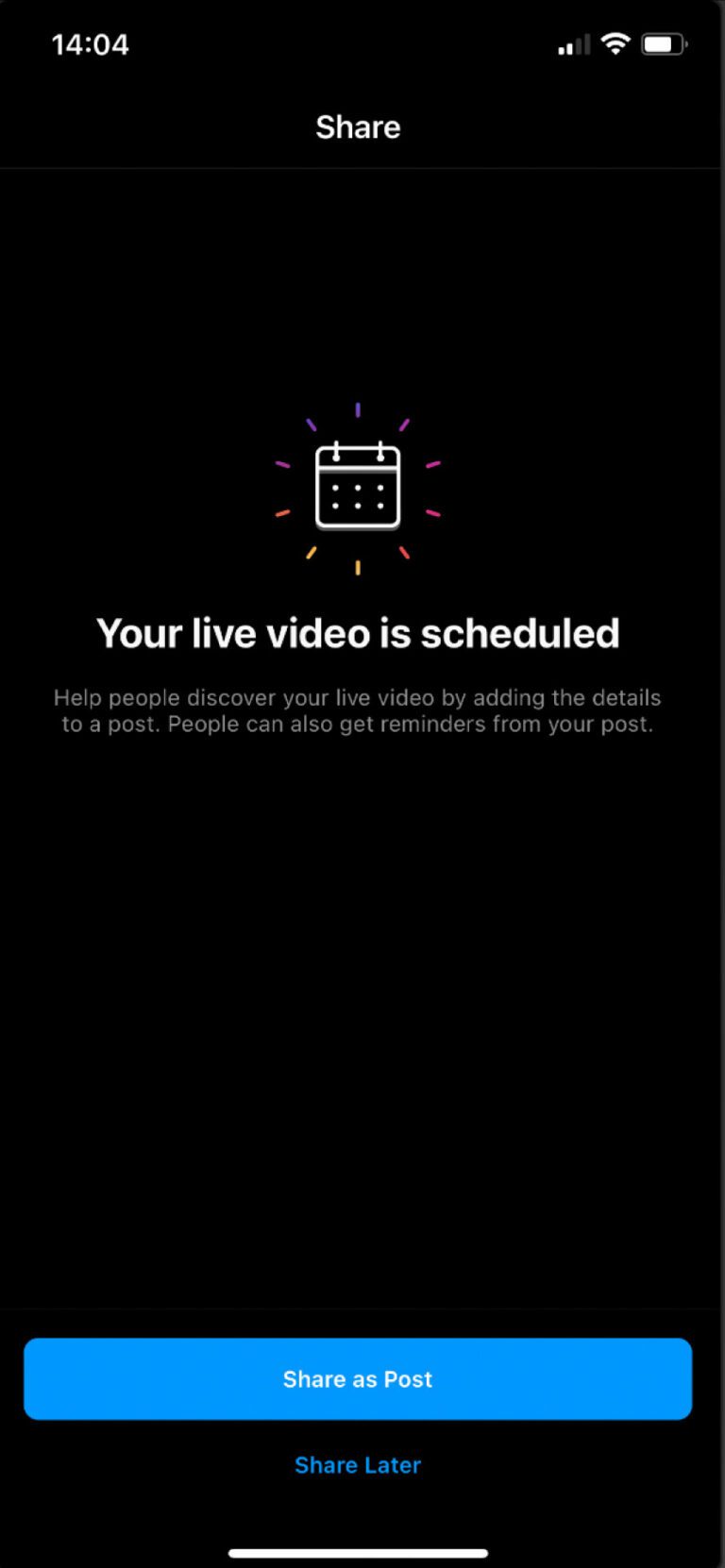A smartphone screenshot showcases the interface for scheduling a live video. At the top, the word "Share" is prominently displayed. Below it, an icon resembling a calendar is surrounded by colorful, radiating lines, reminiscent of fireworks. Directly underneath, a message reads, "Your live video is scheduled." Subtext below the message advises: "Help people discover your live video by adding the details to a post. People can also get reminders from your post."

At the bottom of the screen, a blue button labeled "Share as post" is visible, with a secondary option, "Share later," in blue lettering just beneath it. The top left corner of the screen shows the time as 14:04. To the right, three icons represent network status: the signal strength indicates two out of four bars, the Wi-Fi shows three out of three bars, and the battery icon is more than half charged. The background of the interface is black, and all text and icons are in white.